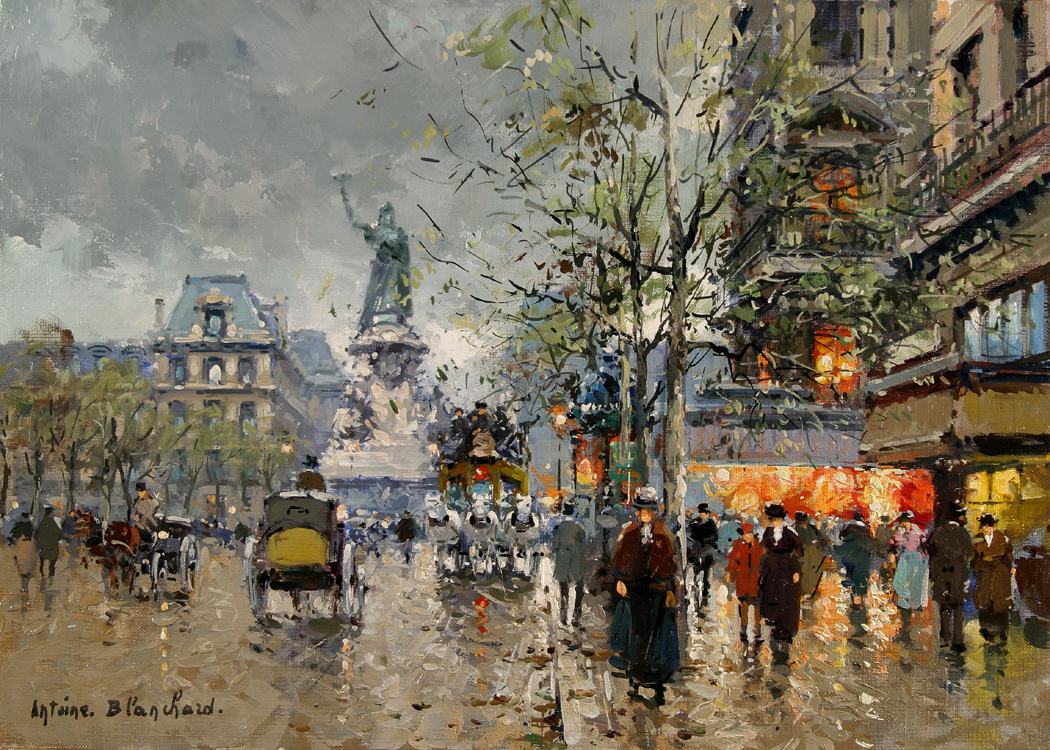This painting by Antoine Blanchard, identifiable by his signature in the lower left-hand corner, captures a bustling city street scene, possibly from 19th-century France. Executed in a textural and somewhat impressionistic style with short, deliberate strokes and dots, the image requires the viewer to let their eyes unfocus slightly to fully perceive its details. On the left side of the painting, a tall four-storied building with arched roofs and an attic looms under a cloudy gray sky. Below the building, trees line the street, their leaves seemingly sparse, suggesting a cloudy or crisp day. A large stone pillar with a statue—its right arm raised—stands prominently, surrounded by the movement of people in horse-drawn carriages passing by on the street below. The scene continues towards the center and right of the canvas, where a line of trees gives way to more structures and a crowded sidewalk filled with shoppers and pedestrians, all depicted in typical 19th-century attire. The detailed yet blurry technique brings the lively urban atmosphere to life, immersing the viewer in the historical ambiance.